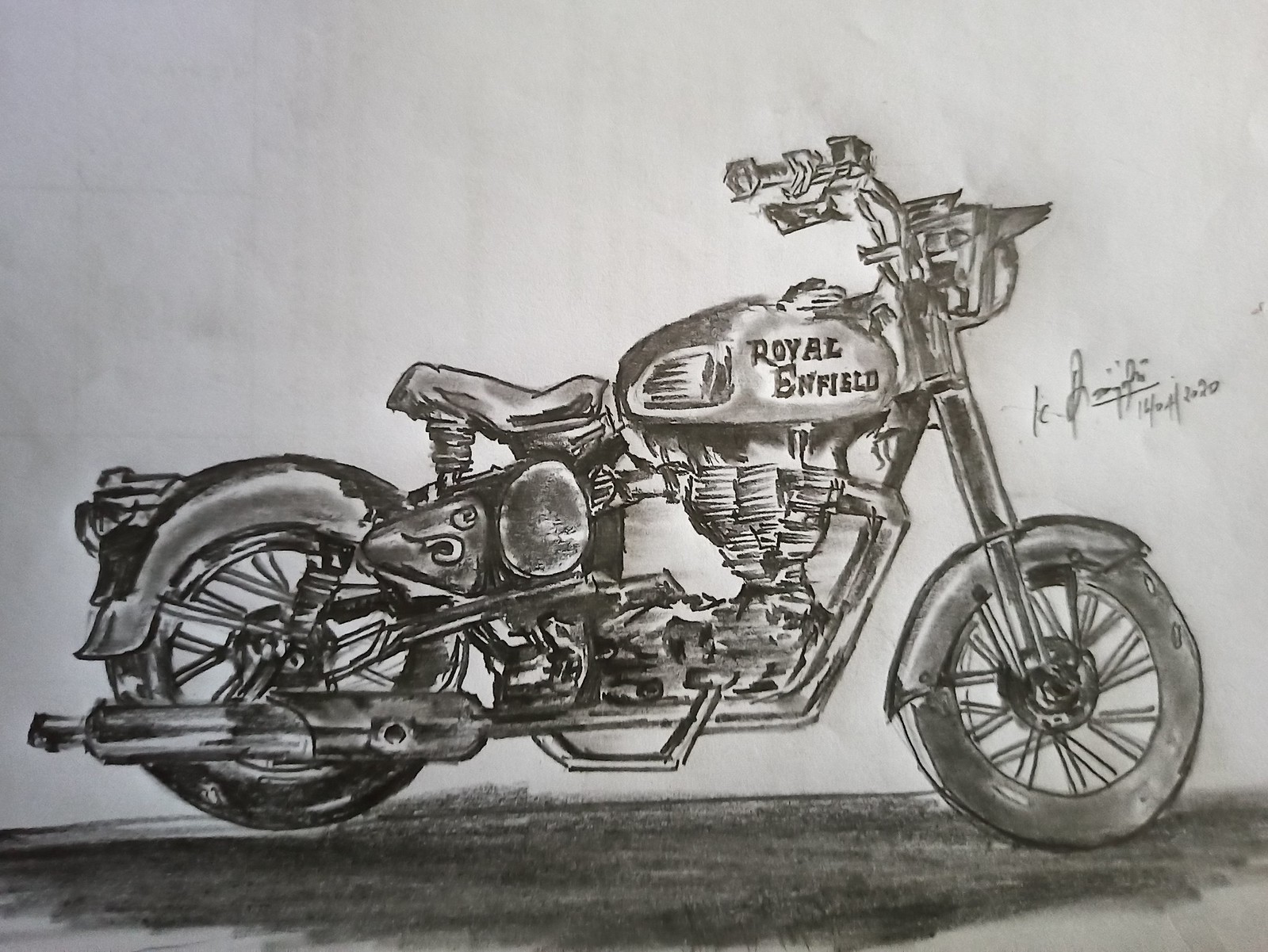This drawing features a meticulously detailed side view of a vintage Royal Enfield motorcycle, prominently centered in the image. The motorcycle appears to be a classic model from the 1930s. The right handlebar is clearly visible, facing the viewer, while the front wheel is positioned to the right and the rear wheel to the left.

The gas tank bears the 'Royal Enfield' logo, distinctly visible to the viewer's side. Directly behind the gas tank, there's a spring-supported seat, typical of the vintage design. The engine is located beneath the gas tank, showcasing intricate mechanical details.

The front wheel, adorned with multiple spokes, has a mudguard covering the top 30% of the wheel. A strut extends downward to a shock absorber, which then connects upward to the handlebar. The rear wheel is partially covered by a fender, which shields about 15% of the tire. At the rear, several lights face backwards, likely indicating brake and tail lights. A gray muffler extends straight back from beneath the engine.

The motorcycle rests on a dark gray road, contrasted by a lighter gray background. The artwork is signed, though the signature is unreadable, with the date "16-04-2020" inscribed below.